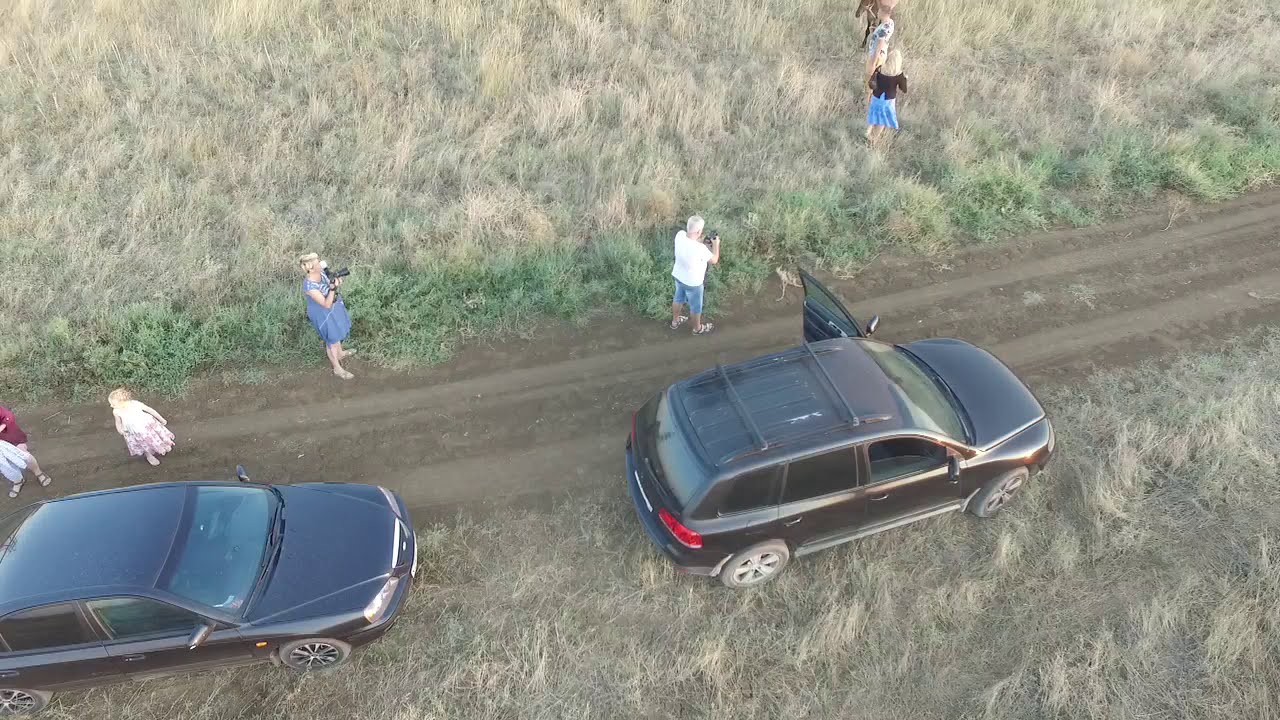The image captures an aerial view of a grassy field intersected by a dirt road that extends from the bottom left corner to the upper right. The dirt road is dark brown where tire tracks mark its surface and lighter brown in untouched areas. On either side of the road, the ground is dotted with long, grayish-tan tufts of grass, alongside patches of yellow and sporadic green grass.

Two cars are parked along the right side of the road. The car more prominently in view, positioned centrally, is a black SUV with silver wheels and an open driver's side door. On top, it is equipped with panels resembling a luggage rack. Behind the SUV is a black sedan.

In total, six people are visible near the cars. In the bottom left corner, a person wearing a red shirt stands next to another individual in a white shirt and pink dress, who is looking backward. Nearby, a person in a blue dress with blonde hair is holding up a black camera. Close to her, a man in a white shirt and blue shorts, wearing sandals, appears to be aiming his camera toward the upper right corner where more people are located. One of these individuals is clad in a black shirt and blue skirt. The overall scene captures the casual dynamics of a small group engaged with their surroundings, set against the backdrop of a rural landscape with distinct tire tracks and varying grass hues.